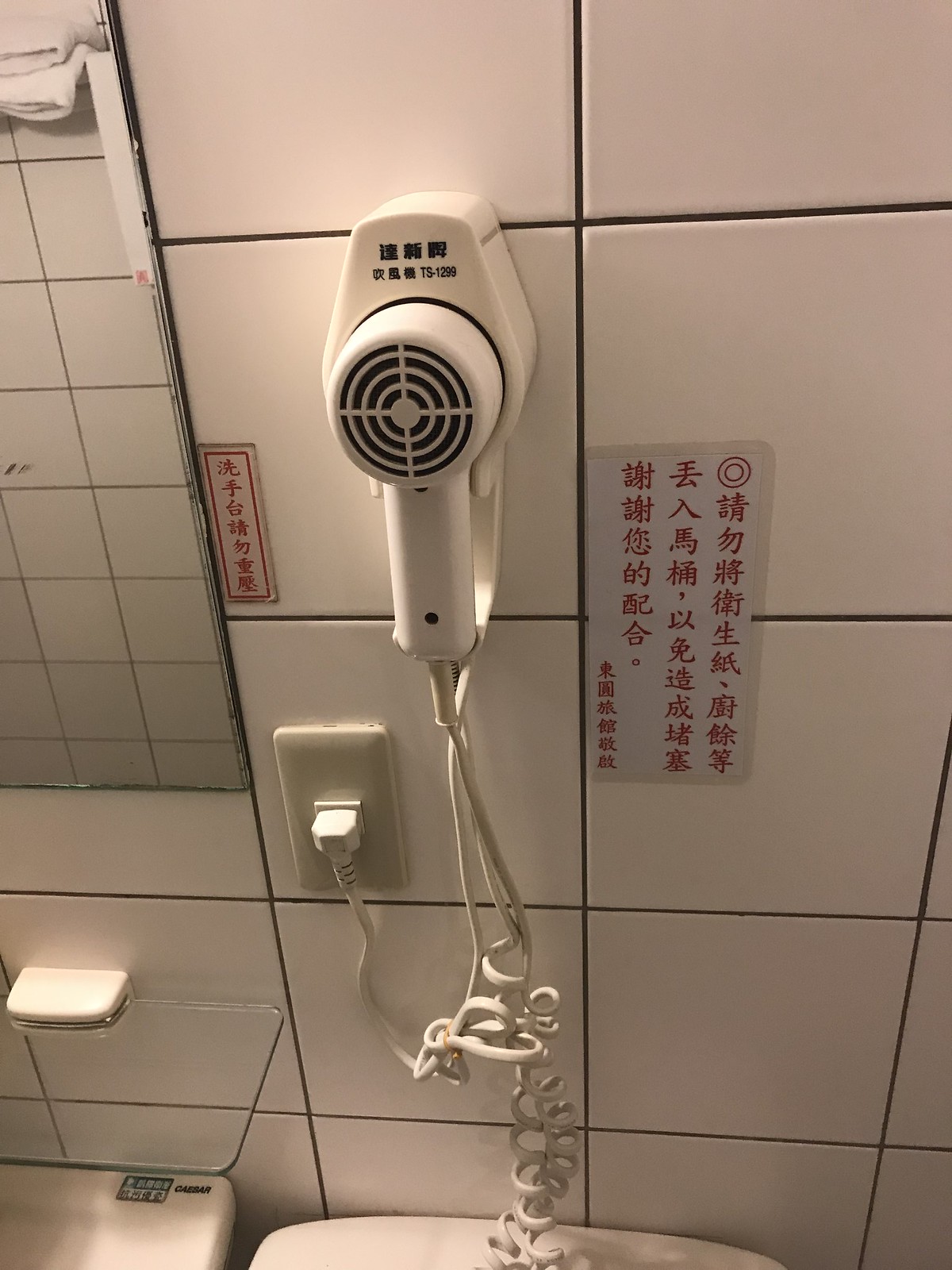The image depicts a pristine white bathroom with checkered white tiles and black grout. Central to the scene is a white handheld hairdryer, plugged into a wall outlet, hanging on a holder that has some black text, including "TS-1299". The bathroom is impeccably organized, featuring a glass shelf, a mirror reflecting the white and black tiled wall, and white towels at the top left corner of the image. Below the hairdryer, there is a white sink with "Caesar" written at the top right, and a white toilet at the bottom of the image. The walls also display two small signs with red Asian writing, one taped near the mirror on the left and the other on the right, detailing some instructions or information.